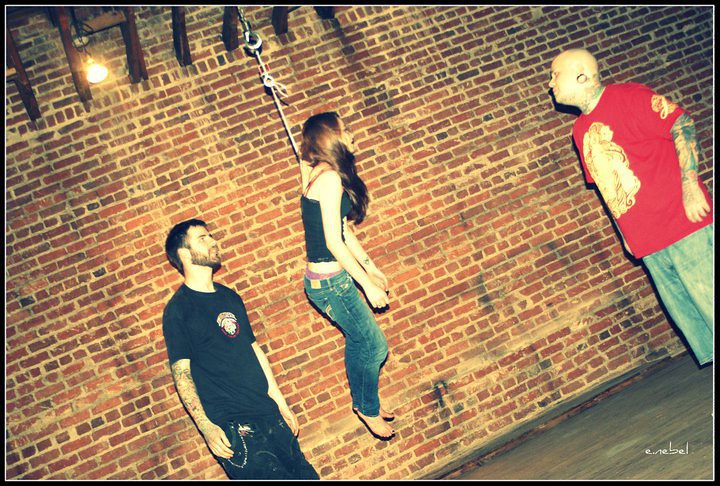In this horizontally aligned rectangular photograph, three individuals are positioned in what resembles an alley against an old brick wall. The scene is illuminated warmly, with hues of orange and yellow. The focal point is a woman with long, straight brown hair, suspended in the air by a thick metal hook attached to a rope around her upper back. She's dressed in a black tank top, jeans, and is barefoot, with a glimpse of her pink underwear visible.

Standing on either side of her are two men, both intently staring at her. The man on the left has short brown hair, facial hair, and a tattooed arm. He is dressed in a black t-shirt with a logo, jeans, and has a chain hanging from his pocket. The man on the right is bald with gauged ears and multiple tattoos on his arms and neck. He wears a red short-sleeved t-shirt with a gold design and denim shorts. The upper left corner of the wall features rusted wooden beams and bars, along with a single light bulb hanging from the ceiling. A watermark is present in the bottom right corner, though it is indistinct.